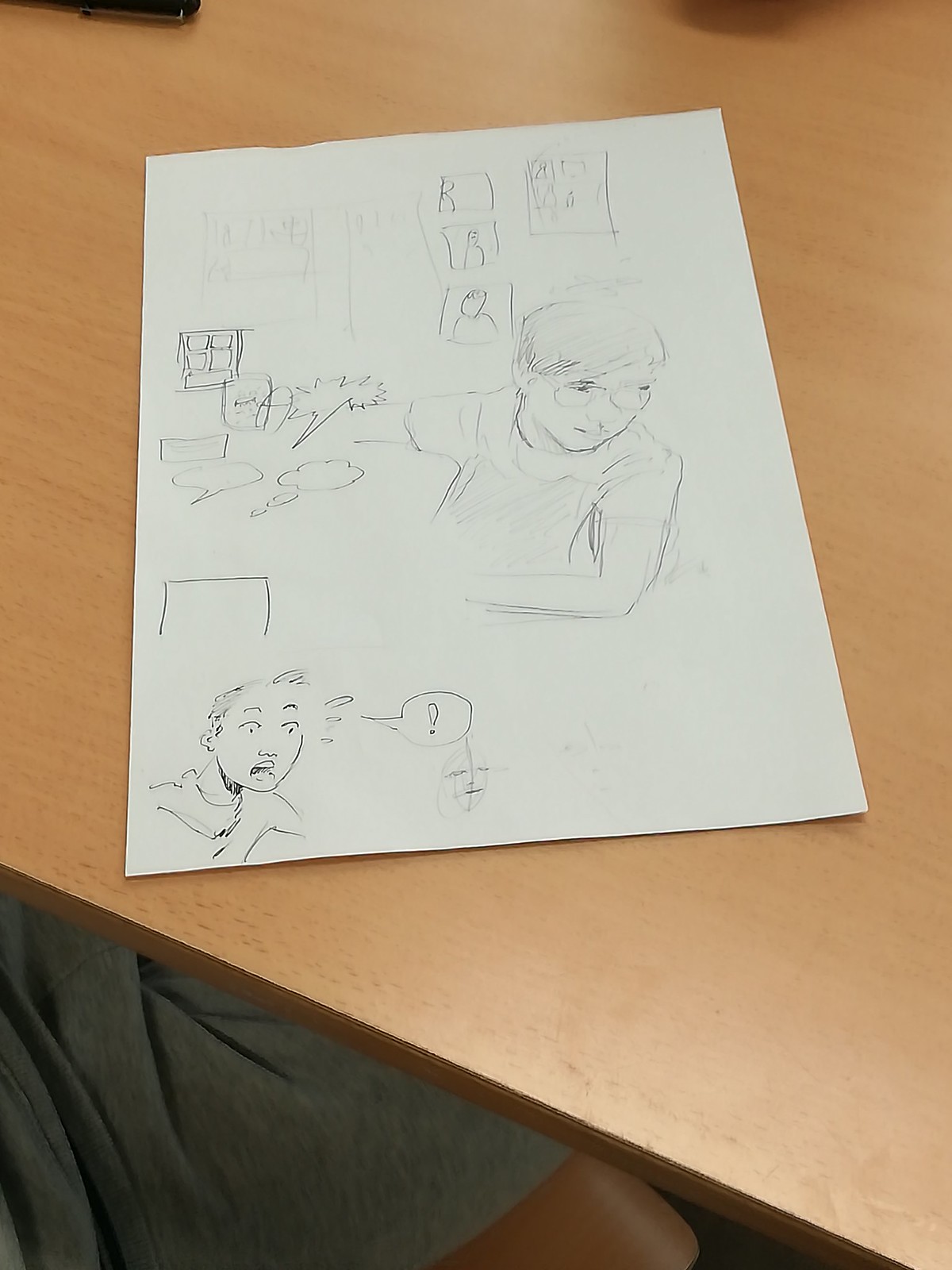On a brown desk in what appears to be a school setting, there is a sheet of white paper featuring a drawing. The lower edge of the desk is visible, along with the partial figure of an individual who is possibly seated there, identifiable by their gray sweatpants. The side of their chair is also visible, displaying a hue similar to the brown of the desk but with a slightly more yellowish tone.

The drawing on the paper seems to be created with a pen, though some lines suggest initial sketches in pencil, given their faded appearance. The artwork depicts two characters: one wearing glasses, who is leaning forward and looking downward contemplatively; the other, positioned at the bottom, exhibits a shocked expression. To emphasize the surprise, a speech bubble with an exclamation point hovers near the shocked character's face.